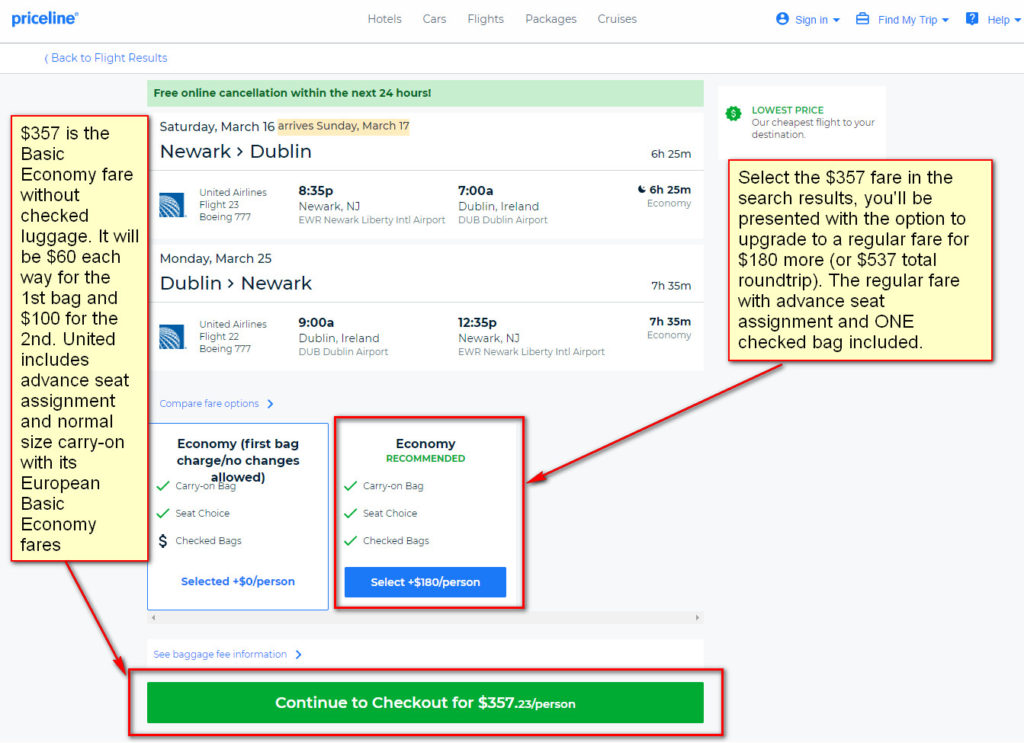The homepage of Priceline is prominently showcased with a clean design and detailed information. 

- **Top Header:**
  - The top inch of the page is white. At the top-left corner, the Priceline logo is boldly displayed in blue. On the right side of the header, there is a small blue text reading "Back to flight results."

- **Navigation Menu:**
  - Centrally positioned, there is a black navigation bar listing options: "Hotels," "Cars," "Flights," "Packages," and "Cruises."

- **Right Sidebar:**
  - From right to left, there are several blue icons and text:
    - "Help" in blue text.
    - A blue square featuring a white question mark symbol and the text "Find My Trip," accompanied by a trip icon.
    - A "Sign In" option with a profile icon next to it.

- **Content Section:**
  - The content area starts with a light gray background.
  - On the left side, there is a vertical tan rectangle bordered in red containing detailed cost information spread across approximately 12 short lines.
  
- **Trip Details:**
  - Adjacent to the tan rectangle, a horizontal light green banner continues across the top. This banner has a dark green text stating "Free online cancellation within the next 24 hours."
  - Below this, there's comprehensive info about the trip:
    - Departure and arrival locations
    - Dates and times of departure and arrival
    - Total duration of the journey
  - There are two separate trip entries provided.

- **Booking Options:**
  - At the bottom, users can choose between:
    - "Economy" on the left, which includes a first bag charge and no options for changes.
    - "Economy Recommended" on the right, marked with a red rectangle.
  - To the right of these options, another square with a red border contains additional cost details.
  - Below the pricing details, an arrow points towards the choice marked within the red rectangle indicating "Continue to check out for $357.23/person" in white text on a green tab.

This well-organized page layout ensures all essential information for travelers is easily accessible, guiding them step-by-step through the booking process.